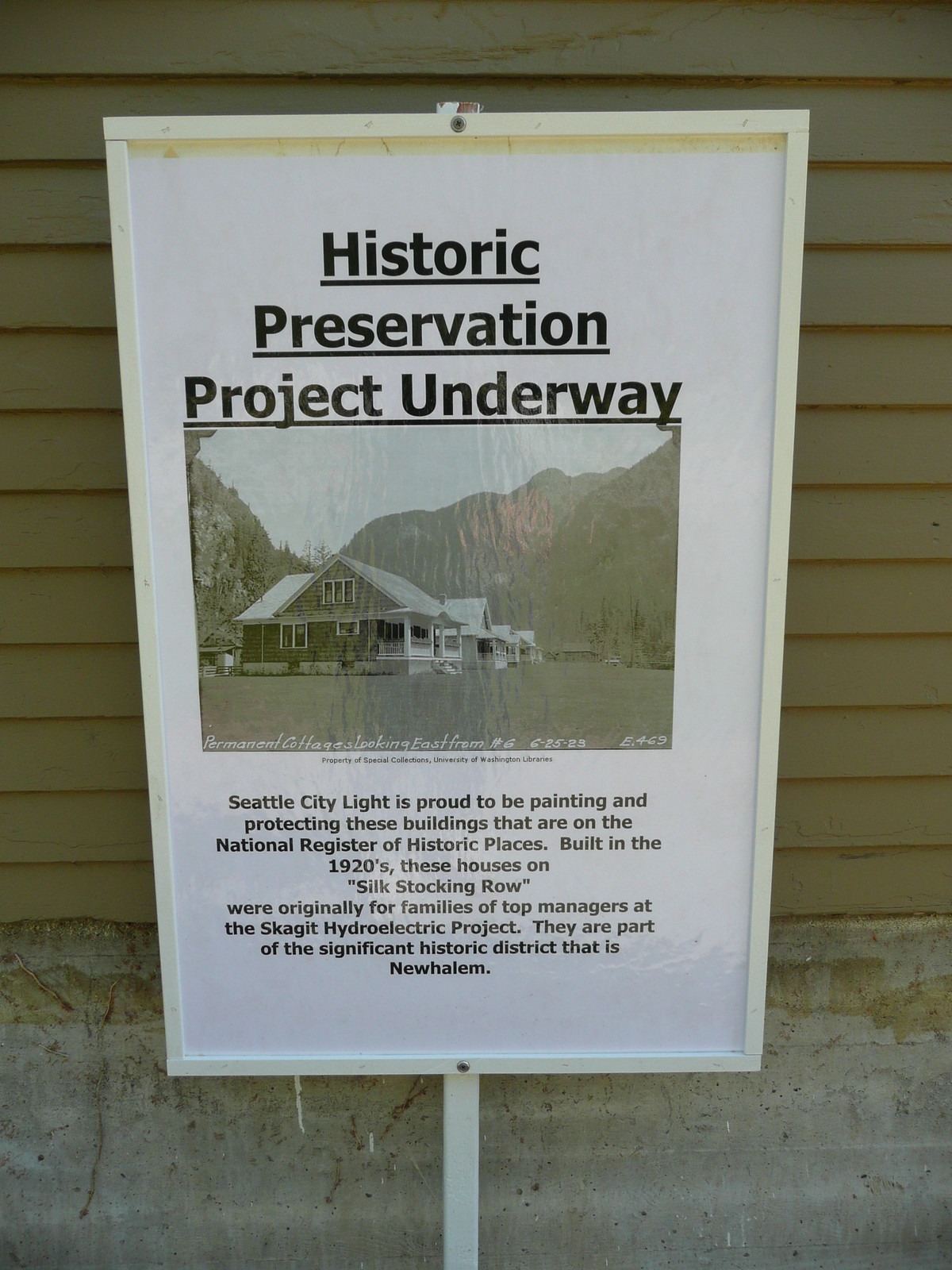The image portrays a rectangular sign mounted on a white metal pole. The photograph captures the sign positioned in front of a house with light brown siding occupying the top two-thirds and a gray stone foundation at the bottom third. The sign itself stands out with its white background and bold black underlined heading at the top that reads, "Historic Preservation Project Underway." Just beneath this heading, a faded black and white photograph depicts a historic row of houses. Following the image, black text states: "Seattle City Light is proud to be painting and protecting these buildings that are on the National Register of Historic Places. Built in the 1920s, these houses on Silk Stocking Row were originally for families of top managers at the Skagit Hydroelectric Project. They are part of the significant historic district that is New Halem." The image was taken outdoors, possibly on a cloudy day, enhancing the nostalgic feel of the historic preservation effort.